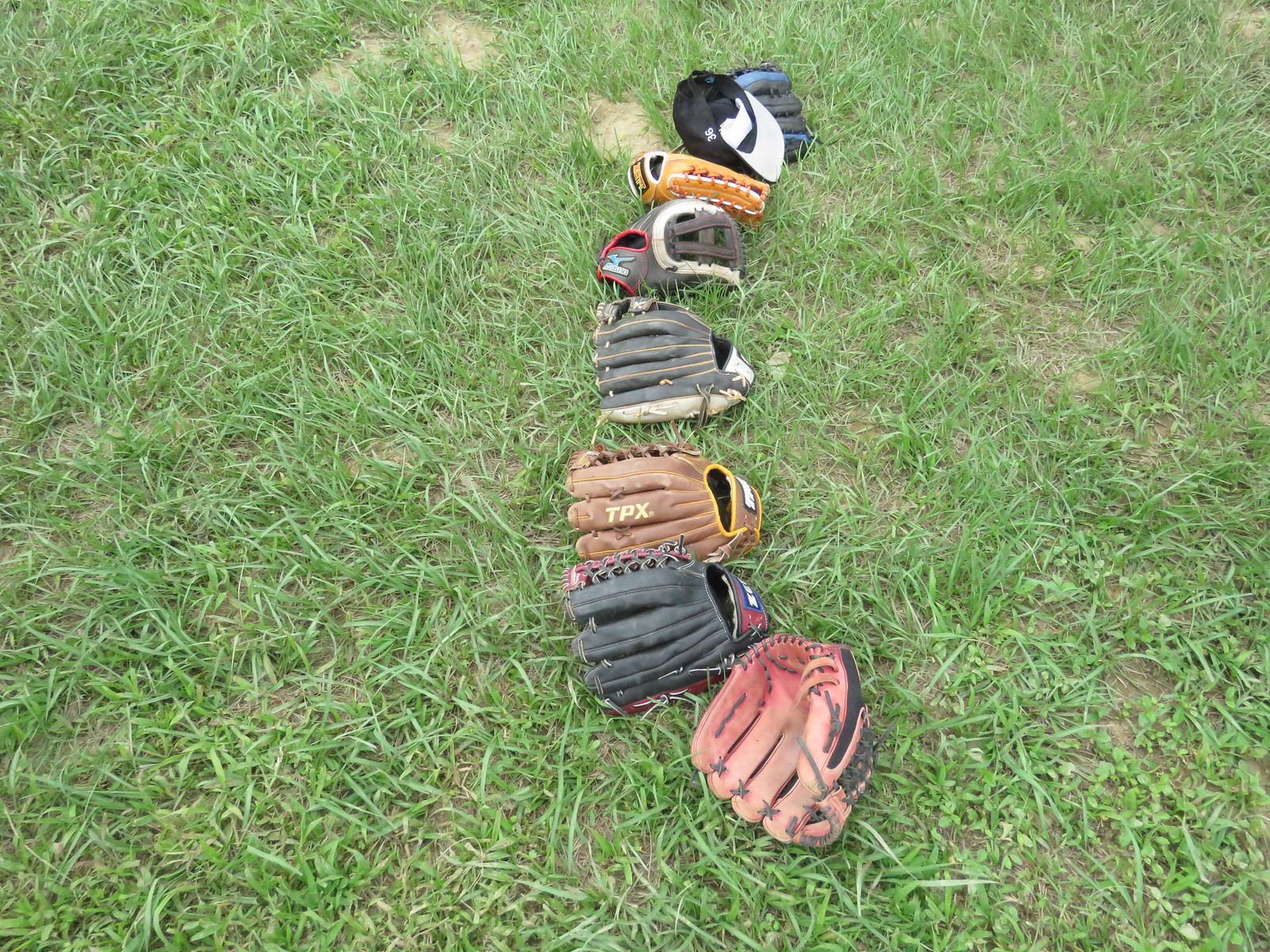In the image, a collection of colorful baseball gloves is artfully arranged on a grassy area. The gloves are laid out at various angles, creating an intricate pattern. To the left and right, several gloves are positioned palm up. At the top, a glove points its fingers to the right, while a glove at the bottom faces its fingers to the left. In the middle, three gloves have their fingers pointing left, and two more at the top have their fingers pointing right. The gloves come in a variety of colors including red, black, brown, and gray, enhancing the visual diversity of the arrangement. The grass beneath them is predominantly green with sporadic patches of mud and soil showing through. The gloves appear to be abandoned momentarily, perhaps after a game, as if the players have left the scene, leaving behind this interesting assortment on the grass.